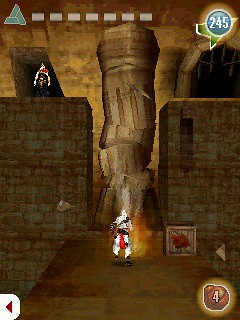A screenshot from a rectangular computer game, possibly designed for mobile platforms, depicts a small character dressed in white clothing standing in the lower middle section, facing away from the viewer. The setting appears to be a crypt or dungeon, characterized by a dominant beige and light brown stone color scheme. Two massive pillars flank the character on both the left and right sides, while a tall column rises up directly behind them, reaching the top of the frame. The background wall behind the pillars and column is a lighter color, adding some contrast. Status indicators for the game are visible in all four corners of the image, providing essential game information.